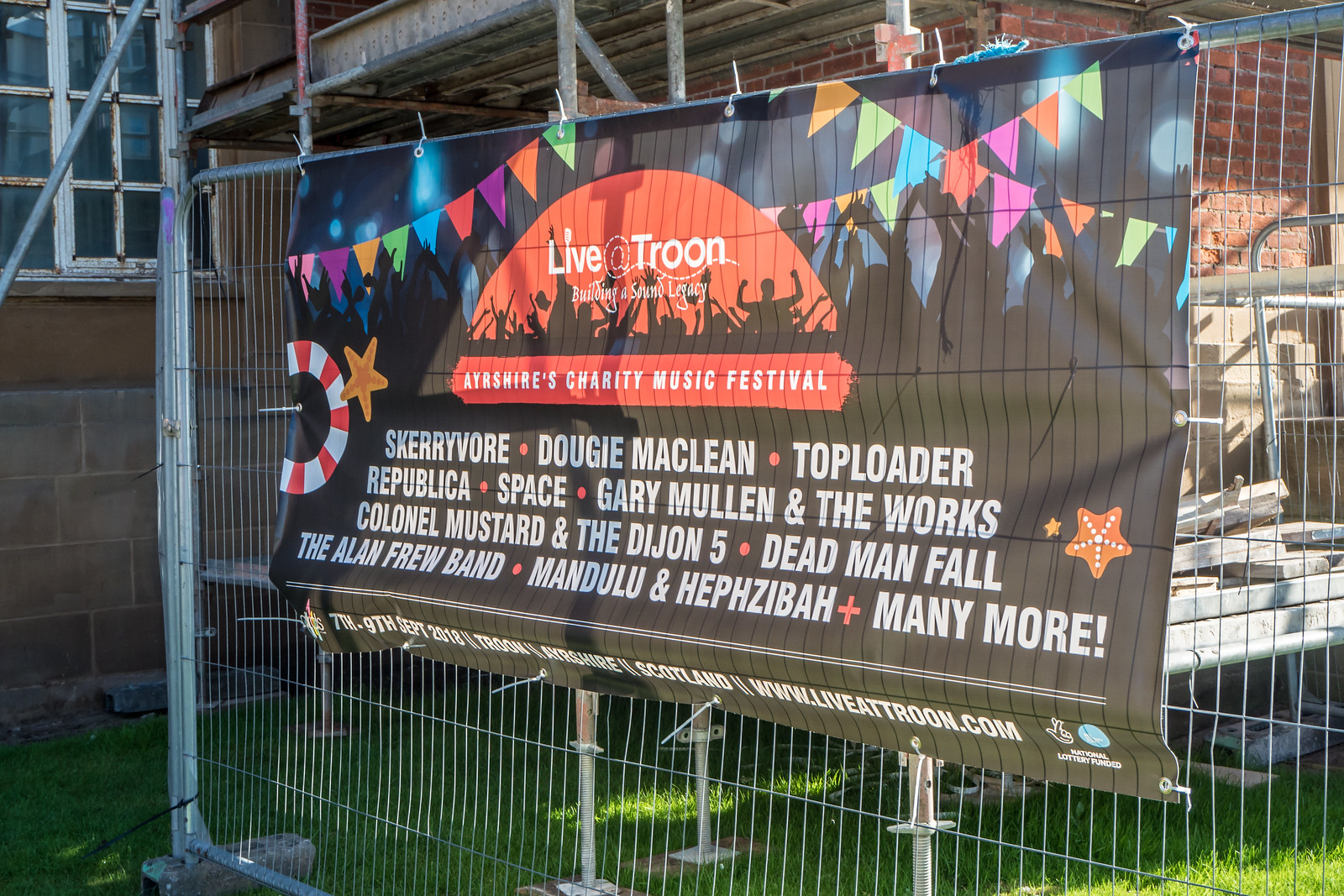A detailed photograph captures a large vinyl banner hanging on wire fencing, angled slightly towards the center-right of the image. The setting is an outdoor, daytime scene, with a backdrop that includes a grassy area below the fence and scaffolding and building materials adjacent to a brick wall with white-paned windows. These windows reveal no interior details. 

The banner prominently reads "Live at Troon," announcing ISHAR's Charity Music Festival. Featured artists include Scary Vore, Dougie McLean, Top Loader, Republica, Space, Gary Mullen and the Works, Colonel Mustard and the Dijon Five, Dead Man Fall, the Alan Frew Band, Mandulu and Hebzibah, among many others. The bottom of the banner provides further details, stating the event will take place from September 7-9, 2018, in Troon, Ayrshire, Scotland, and is funded by the National Lottery. The festival’s website, www.liveattroon.com, is also displayed. The banner is colorfully decorated with shades of orange, yellow, light green, black, white, red, purple, pink, brown, beige, gray, green, dark green, and tan. The design includes silhouettes of a festival crowd along with life preservers and starfish, hinting at a beach party theme.